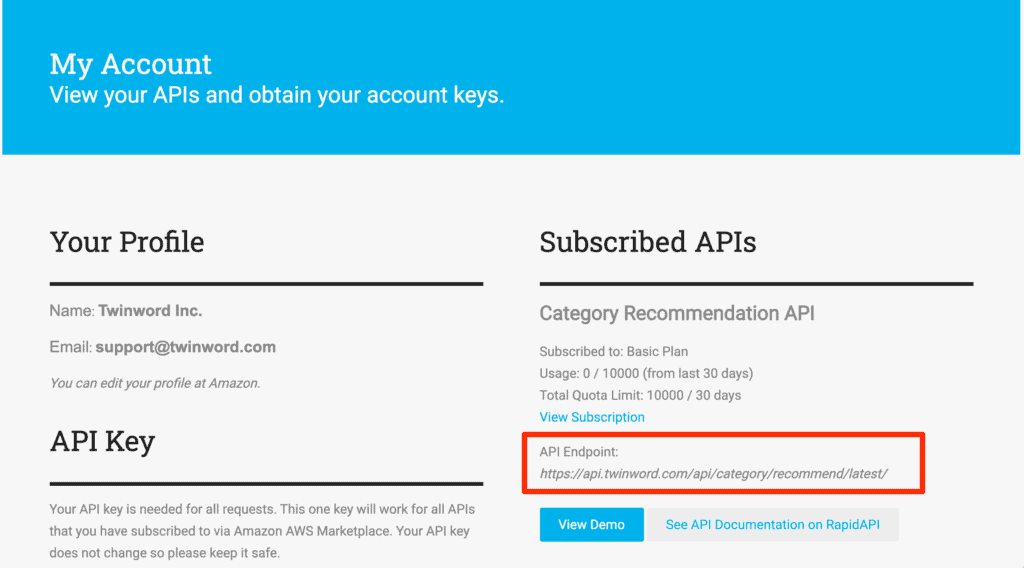Account Details Panel for APIs and Account Keys

At the top of the panel, there is a thick blue header bar that spans the entire width and prominently displays the text "My Account." Below the header, detailed sections are presented to manage APIs and account keys, primarily geared towards services subscribed via the Amazon AWS Marketplace.

On the upper left side, key account information is listed:
- **Profile Name:** Twinworld, Inc.
- **Email:** support@twinworld.com
- There is an option to edit your profile at Amazon, suggesting that the API keys are actually for Amazon services.

Under this section, additional details about your API key are provided:
- Your API key is essential for all API requests.
- One API key works across all APIs subscribed via Amazon AWS Marketplace.
- The key is permanent; hence, it is critical to keep it secure.

In the next column to the right, subscription details are displayed:
- **Category:** Recommended APIs
- **Plan:** Basic 
- **Usage:** 0 of 10,000 requests for the last 30 days
- **Total Quota Limit:** 10,000 requests per 30 days
- A clickable blue text link to "View Subscription"

Below this section, enclosed in a red-bordered box, is the API Endpoint:
- A full URL is displayed showing the API endpoint address.

At the bottom of the panel, two buttons are available for additional actions:
- A light blue button labeled "View Demo"
- A light gray button with light blue text, labeled "See API Documentation on RapidAPI"

This detailed layout ensures easy access to all necessary API and account information for efficient usage and management.